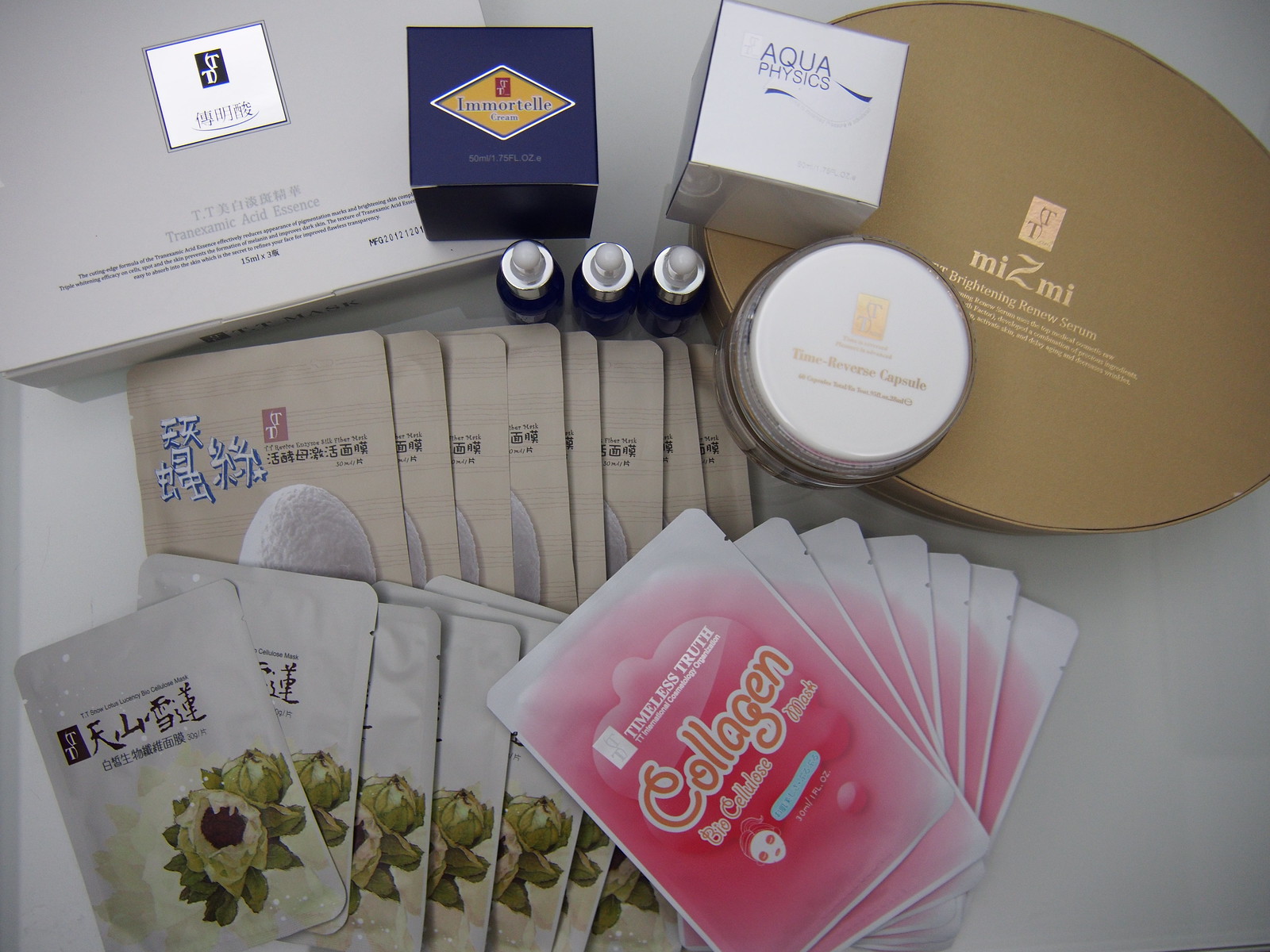The photograph captures an array of diverse skincare products meticulously arranged on a clean, white table, forming an intricate, multi-layered display. Starting from the top left, a large rectangular white box stands prominently, although its lettering remains indiscernible. Perched on the lower right-hand corner of this box is a smaller, nearly cubic box featuring a yellow diamond-shaped label with blue text, though the specifics of the writing are unclear.

Directly to the right of this smaller box, another white cubic box with blue lettering reading "Aquaphysics" is positioned. This cube rests on top of an oval brown box labeled "Ms. Me," with the design incorporating a lowercase 'm', and 'i' bracketing an uppercase, stylized 'Z', all in a lighter brown shade than the box itself. Atop the oval box lies a round container adorned with a white label and peach-colored writing, which is unfortunately too blurry to decipher.

Moving downward, three navy blue glass bottles featuring eyedropper lids are lined up neatly. Below this trio, eight flat packets, cream-colored and bearing a white design resembling soap, are displayed. The labels on these packets are written in an Asian language, combining blue, white, and black text.

To the lower left, seven flat packets can be seen, each adorned with a greenish flower featuring a light green center, similarly labbeled in an Asian language using black text. On the right side of the display, six rectangular packets of collagen boast a predominantly pink hue with white borders. These packets are flat, each featuring a small image of a lady at the bottom and the word "collagen" prominently written in orange, set against a white background with a white border. 

Overall, the composition showcases various skincare products, blending different shapes, colors, and textures, all thoughtfully arranged against the pristine backdrop of a white table.